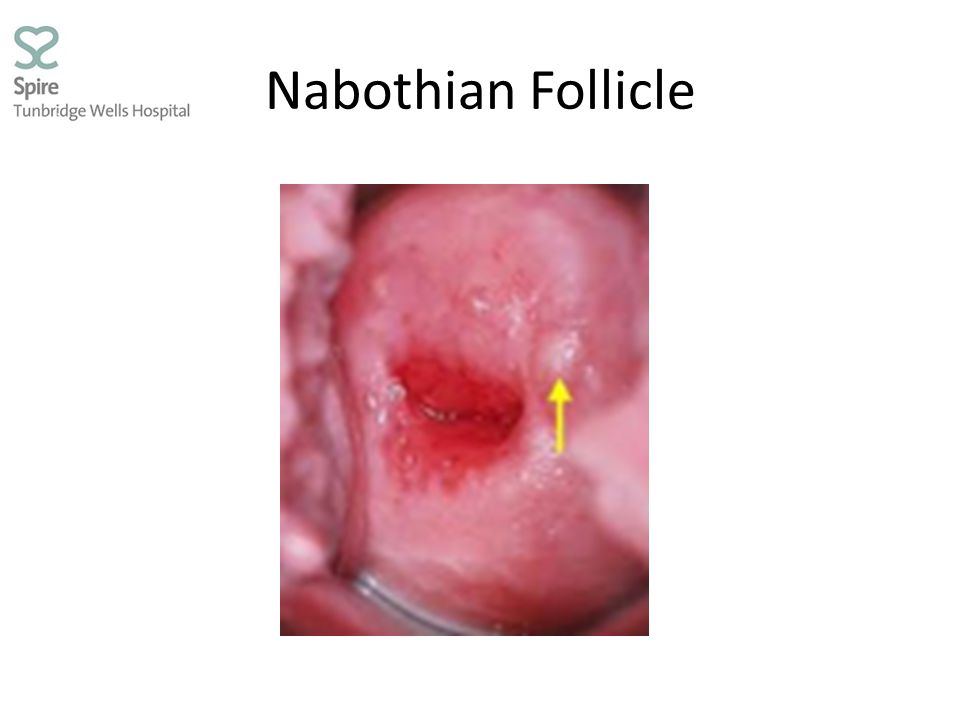The image showcases a highly detailed, up-close photograph of what appears to be the inside of the human body, specifically a Nabothian follicle. The photograph, set against a stark white backdrop, is marked with text indicating its source from Spire Tunbridge Wells Hospital, accompanied by a heart symbol. The primary focus of the image is a pink, fleshy, somewhat gummy area of tissue, prominently featuring a raised, white, pimple-like bump identified by a small yellow arrow. This bump is presumably the Nabothian follicle. In the background, a reddish-pink blur suggests additional organic tissue. The scene may be intended for an educational context, possibly within medical training or surgical reference materials, emphasizing detailed anatomical features.